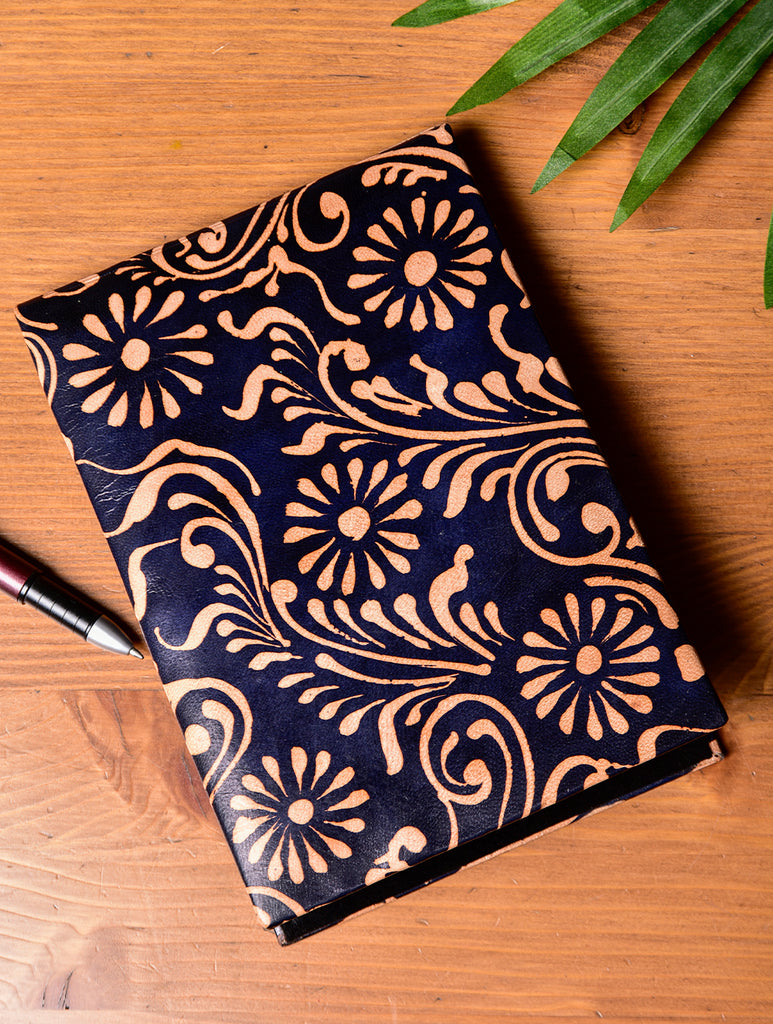A richly detailed image showcases a tilted dark blue journal with light peach flowers and intricate designs on its cover. The background color of the notebook is unmistakably dark blue, adorned with five delicate peach-colored flowers. One flower is centrally placed while the other four are positioned in each corner. The central flower is surrounded by leafy designs. The journal, which has no text on its cover, rests on a medium brown wooden surface, notable for its pronounced grain. To the left side of the image, a partially visible pen with a metal gray tip, a black plastic section, and a red main body sits close to the journal. In the top right corner of the image, partial leaves can be seen, adding a touch of natural elegance to the scene. The journal’s cover hints at a luxurious texture, and the wood surface below it complements the overall warm and aesthetically pleasing composition.